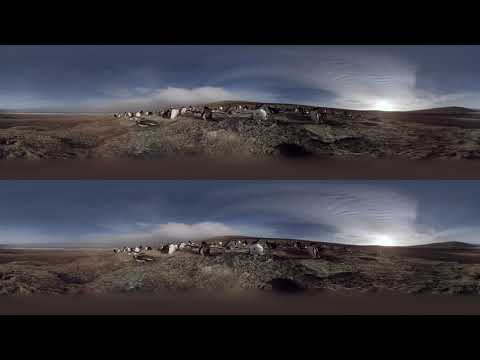This small, horizontally rectangular image is framed by thin black bands at the top and bottom. The internal content consists of two nearly identical, low-resolution, panoramic landscape shots stacked vertically. 

Both panoramas capture a sunset scene, portraying a partly cloudy sky with a gradient from dark blue at the top to lighter tones near the horizon, where scattered white clouds are visible. The horizon runs through the middle of each panorama, dividing the frame into a sky above and a ground section below.

The terrain features a mix of barren fields, rocky ground, and large boulders, with a notable absence of lush greenery. The hillside hosts a few scattered buildings, including white structures that stand out, though most of the buildings appear indistinct due to the image's dark lighting and low resolution.

Together, these elements create a composite image wider than it is tall, maintaining a 16x9 orientation reinforced by the black borders. This visual format emphasizes the repetitive, panoramic nature of the scene, capturing a distant cityscape set against a dramatic dusk sky.